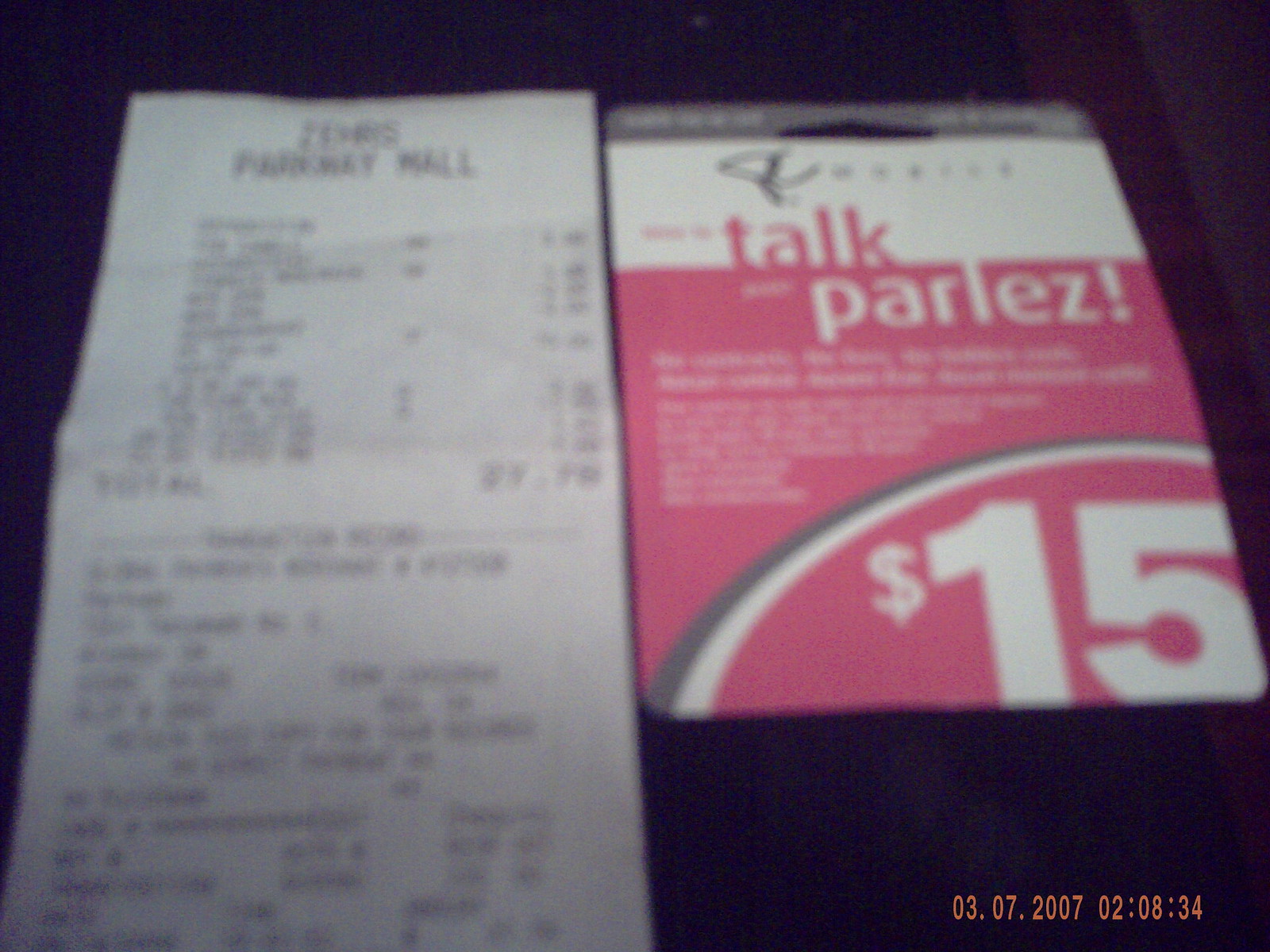The photograph captures an angled view of a receipt and a gift card laid side-by-side on a blue background, with a date and time stamp in the bottom right corner reading "03, 07, 2007, 02, 08, 34." The receipt is positioned on the left and appears to be from a mall, though the top two words are indistinct. It lists several blurry items and shows a total amount. The gift card on the right features a gray border at the top with a cutout for hanging in a retail display, followed by a white section and then a dark pink section. The white section contains the word "R" handwritten in pink and prominently displays the word "TALK" in red. Below, in the dark pink section, the word "PARLEZ" is printed in white. At the bottom right corner of the gift card, "$15" is clearly marked in white, with a subtle curved design in white and gray above the "$15."